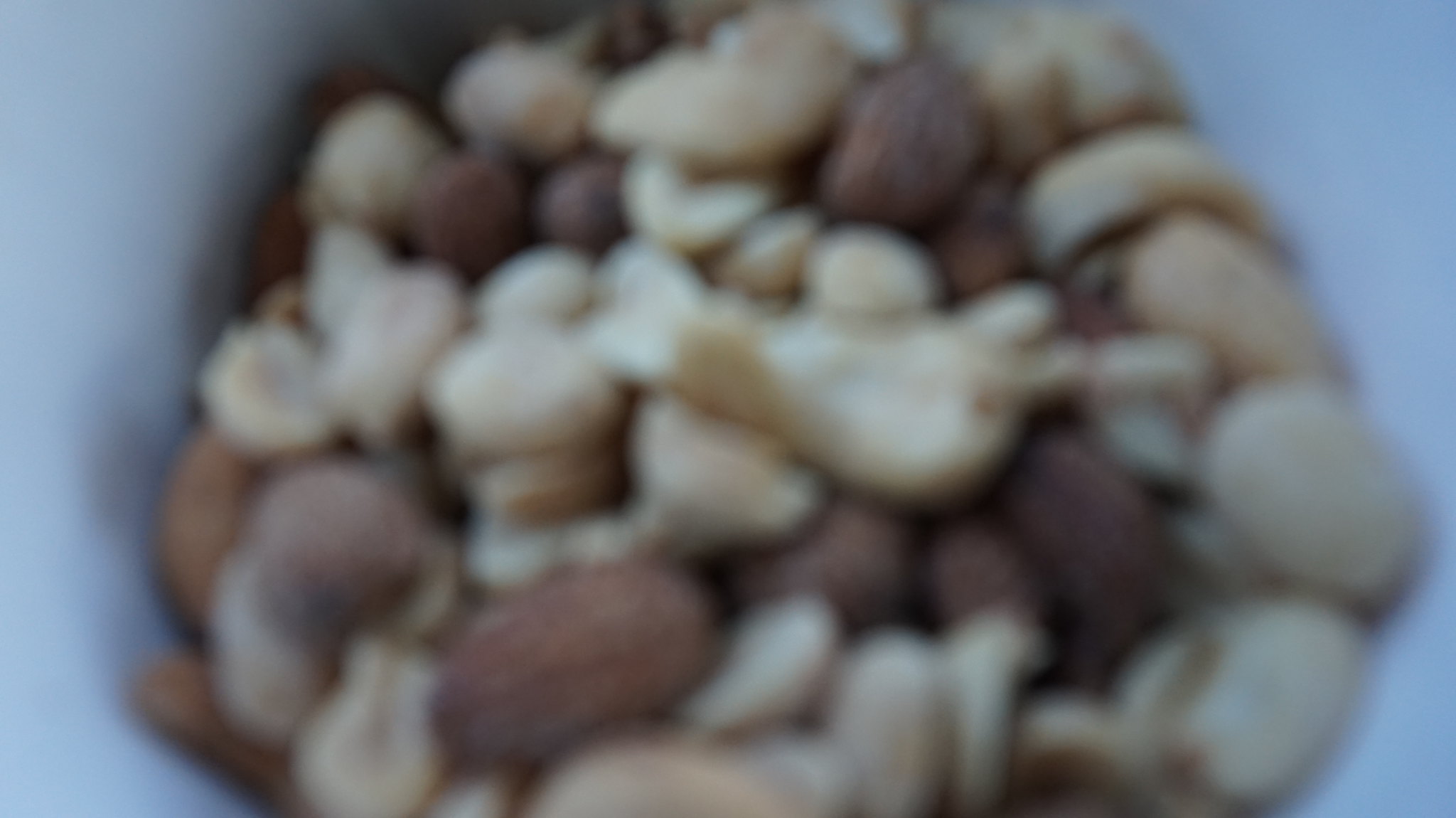The image depicts an elongated rectangular frame with a predominantly white or very light gray background. Central to the composition, occupying the majority of the frame, is a slightly blurry close-up of an assortment of nuts. These nuts appear to be contained in a circular arrangement, likely within a cup or bowl, spilling slightly over the edges of the container. The assortment includes various kinds of nuts such as pecans and peanuts, exhibiting a mix of colors from light tan or whitish peanuts to darker and lighter shades of brown. The nuts seem evenly distributed, though there is a slight predominance of the lighter-colored peanuts. The scattered nuts against the neutral background create an interesting visual contrast, suggesting the possibility of this being a simple depiction of mixed nuts rather than a trail mix, which would typically include other ingredients.